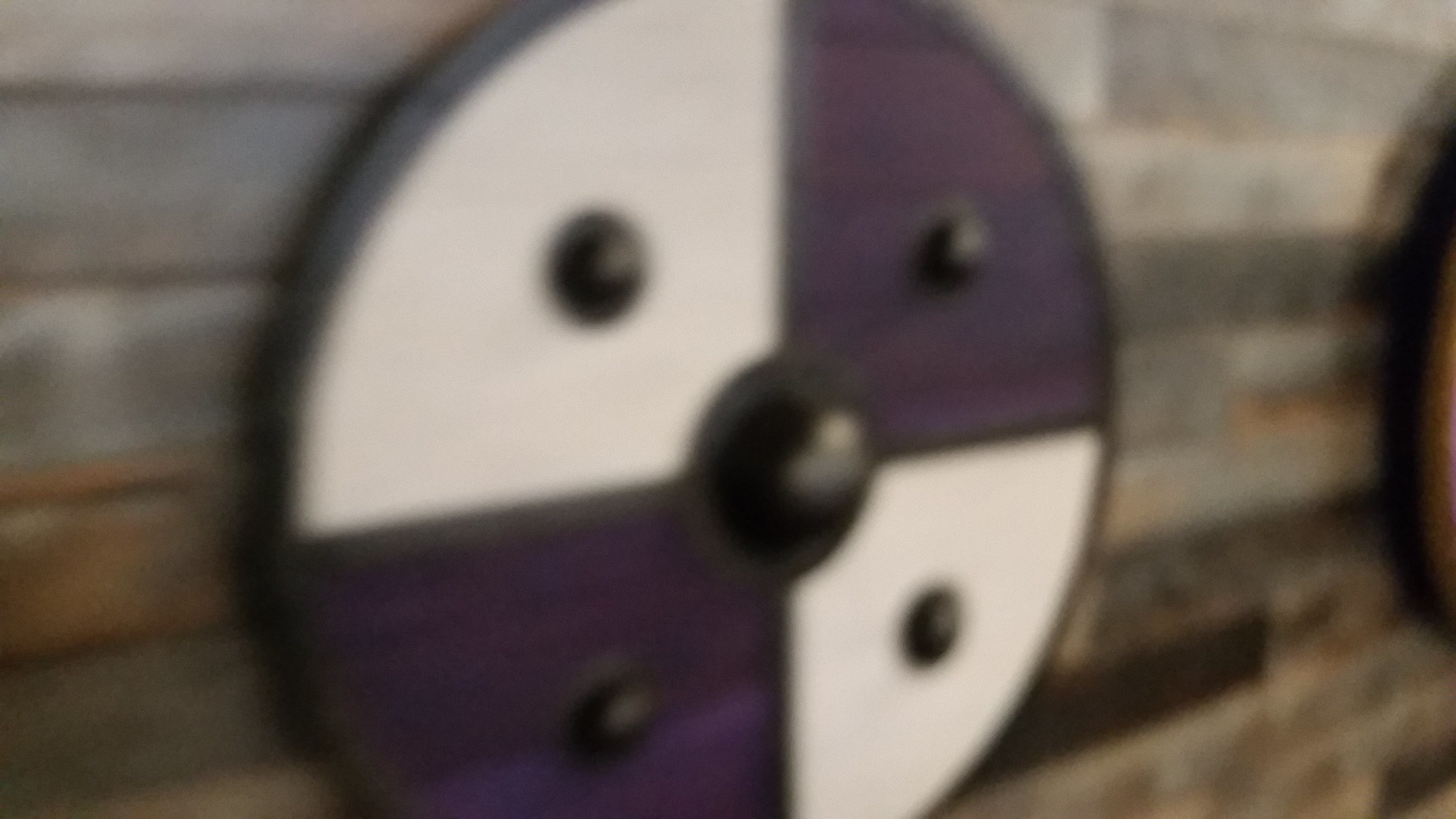A meticulously crafted round shield hangs on a rustic wooden wall composed of varying shades of gray, white, brown, and reddish wood arranged in horizontal slats. The shield features a symmetrical design with alternating blue and white triangular sections converging at the center. Each of the blue and white segments is adorned with a prominent black dot. A bold black cross extends from the central point towards the edge, creating a striking contrast against the colored sections. At the heart of the shield lies a large, protruding black nub, adding depth and focus to the overall appearance. The shield's rim is also lined in black, providing a cohesive frame that complements its intricate design.